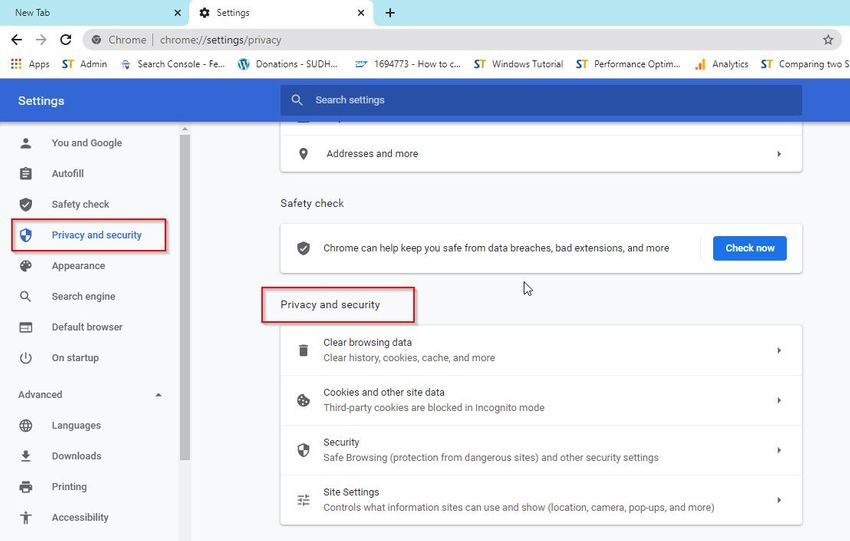The screenshot displays a browser window with a gray background, featuring two tabs labeled "New Tab" and "Settings." The URL in the address bar reads "chrome://settings/privacy." 

The browser interface includes several bookmarked items such as "Apps," "st admin," "Search Console," "fe...," "donations," "sudh...," "how to," "c...," "st windows tutorial," "st performance," "optim...," "Analytics," "st comparing to," and a few others that are partially obscured.

On the left-hand side of the settings page, a vertical menu lists various sections: "You and Google," "Autofill," "Safety Check," "Appearance," "Search Engine," "Default Browser," "On Startup," "Advanced," "Languages," "Downloads," "Printing," "Accessibility," "Addresses and More," and "Safety Check."

Highlighted in the settings menu is "Privacy and Security," surrounded by a red rectangle. This section offers options such as "Clear browsing data," "Cookies and other site data." Additionally, there's a blue rectangle labeled "Check now" in white, situated under a note stating, "Chrome can help keep you safe from data breaches, bad extensions, and more."